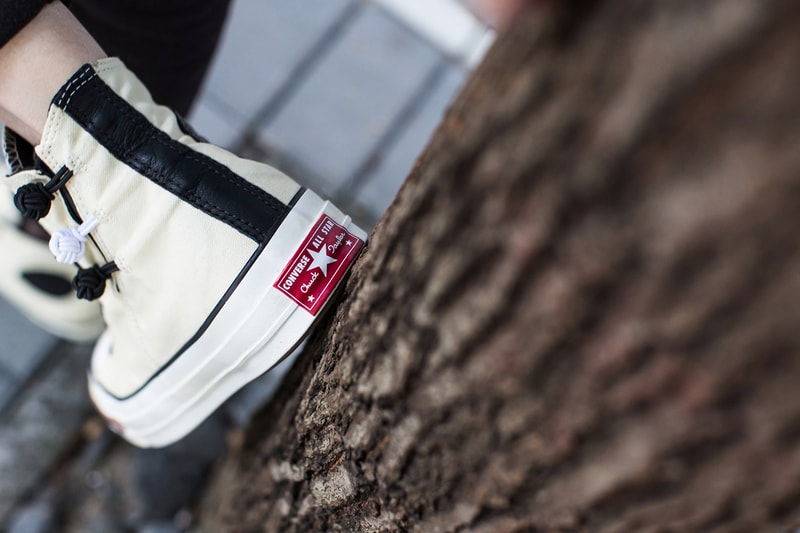This is a detailed angled close-up view of the back of a high-top Converse tennis shoe captured in a color photograph. The shoe is worn by a person and rests on a log, which juts toward the viewer at an unusual angle, giving the sneaker a somewhat sideways appearance. The heel of the shoe is in sharp focus, prominently displaying a red label with the white Converse All-Star logo and text, along with a white star in the center. The shoe itself is white, with a black stripe running down the heel, terminating where the heel meets the sole. The sole is white rubber. The shoelaces are crafted from cord and tied in a ball knot on the left side. The background features an out-of-focus gray paneled house wall. Most of the picture is out of focus except for the shoe and the part of the log it rests on.